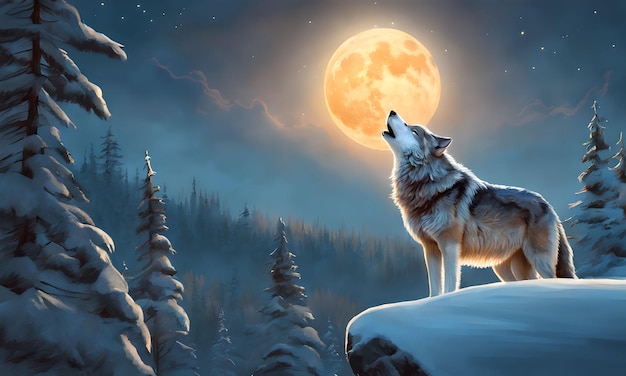The image is a smooth, detailed illustration, possibly a digital or painted artwork, depicting a nocturnal winter scene with a gray wolf howling at a glowing moon. The wolf, positioned on a snow-covered cliff ledge, has its head and snout raised towards the sky, emphasizing its howl. The full moon, which appears to be a radiant orange-yellow, illuminates the foggy, dark-blue night sky. Surrounding the wolf is a landscape filled with snow-dusted evergreen pine trees, creating a serene yet haunting atmosphere. The background reveals a fog-enshrouded mountain landscape, adding depth to the scene. Tiny white dots, representing stars, dot the sky above the moon, contributing to the overall mystique of the wintry night. The illustration itself is rectangular, approximately 4 inches wide by 3 inches high, capturing the beauty and isolation of nature in a cold, dark, winter night.